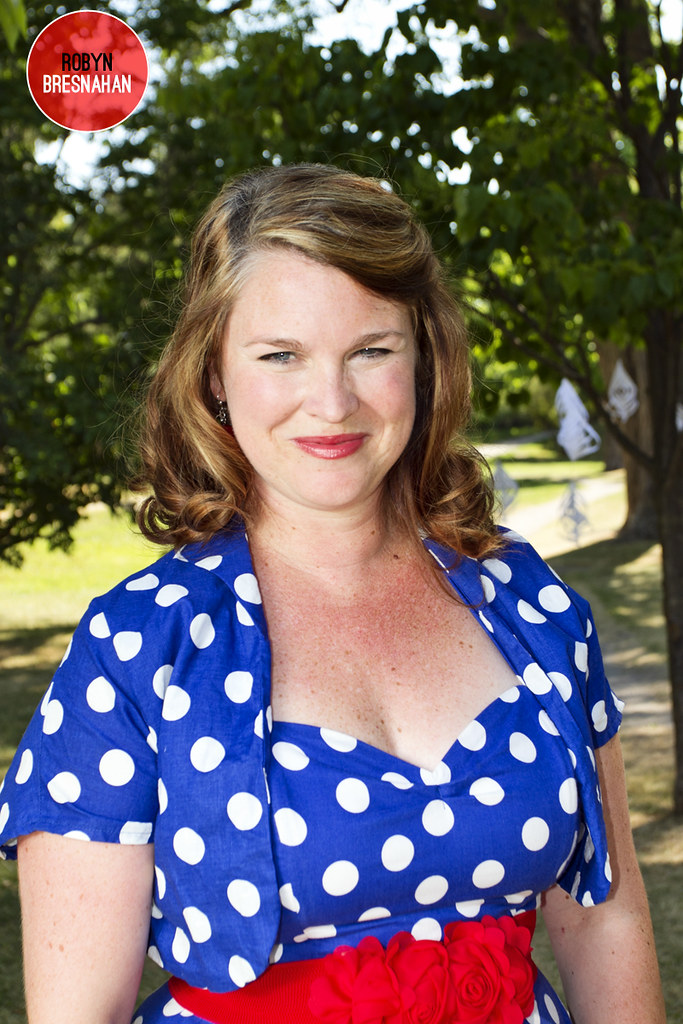The color photograph captures a smiling woman, depicted from the waist upwards, dressed in a vibrant blue dress adorned with white polka dots. Complementing her ensemble is a matching short-sleeved blue coat with the same polka dot pattern. At her waist is a distinctive red belt embellishing the front with red roses. She wears red lipstick that accentuates her bright smile and blue eyes, while her blonde-tinted brown hair, parted on the right, flows naturally over her shoulders. Dangling earrings add an element of elegance to her look. The background portrays a serene park setting, with a tree decorated with multiple white ornaments situated to the right, and a cement walkway centrally located and stretching behind her. To the left of the walkway is a green expanse of grass. The sunny ambiance is underscored by the presence of shadows and light gives a sense of warmth to the scene. In the upper left corner, a red watermark with the name "Robin Presnahan" appears, subtly marking the photograph. The image is bathed in natural light, subtly highlighting the woman’s freckles and hint of sunburn on her chest.